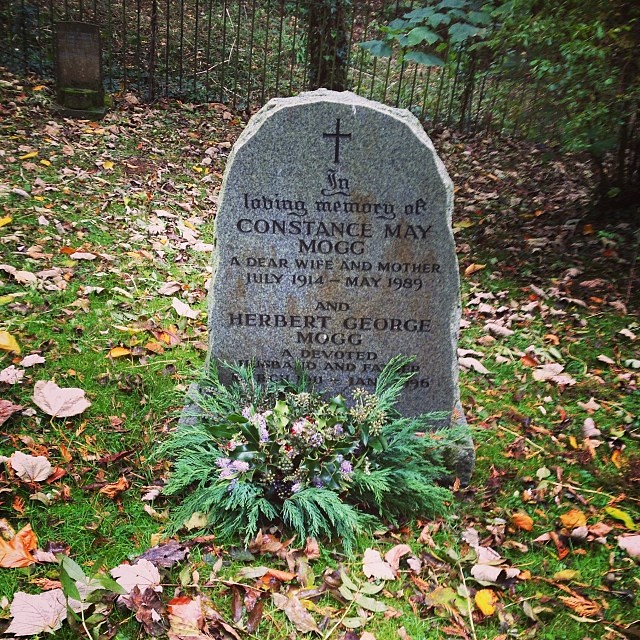The color photograph features a gray granite tombstone prominently placed at the center of a cemetery. The stone, polished on the front and rough-cut around the edges, has a dome-shaped top reminiscent of a bullet pointing skyward. The surface of the tombstone is speckled with black and other colors. An engraved black cross sits at the top, followed by the inscription: "In loving memory of Constance May Mogg, a dear wife and mother, July 1914 - May 1989" and "Herbert George Mogg, a devoted husband and father." However, the text concerning Herbert is partially obscured by a plant with pine needles and colorful flowers positioned in front of the tombstone. A scattering of dead leaves covers the grass beneath it, while a wrought iron fence and trees with overhanging vegetation form the background. Another tombstone is visible in the upper left corner of the image, adding depth to the tranquil scene.